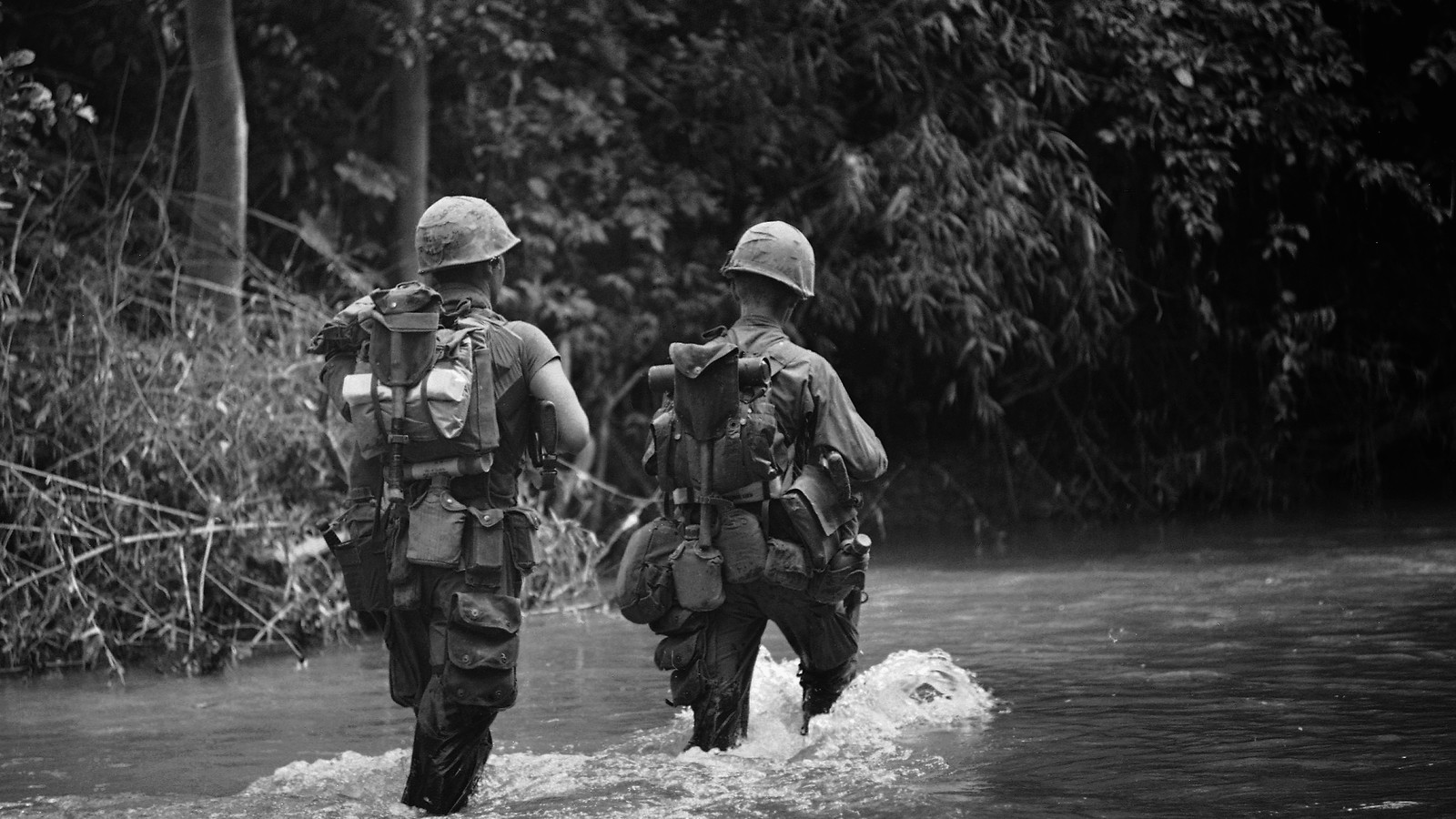In this black and white military photograph, two soldiers, seen from behind, are walking through shallow water that splashes up to just below their knees. Equipped with helmets and carrying substantial tactical gear on their backs, including small shovels and canteens around their belts, they move through the watery terrain. The end of a gun peeks from underneath the right arm of each soldier, confirming they are armed. Both wear dark pants as they navigate this possibly jungle environment, indicated by the dense leaves and tree trunks visible in the background. The image suggests a scene from a military operation, perhaps reminiscent of the Vietnam War.